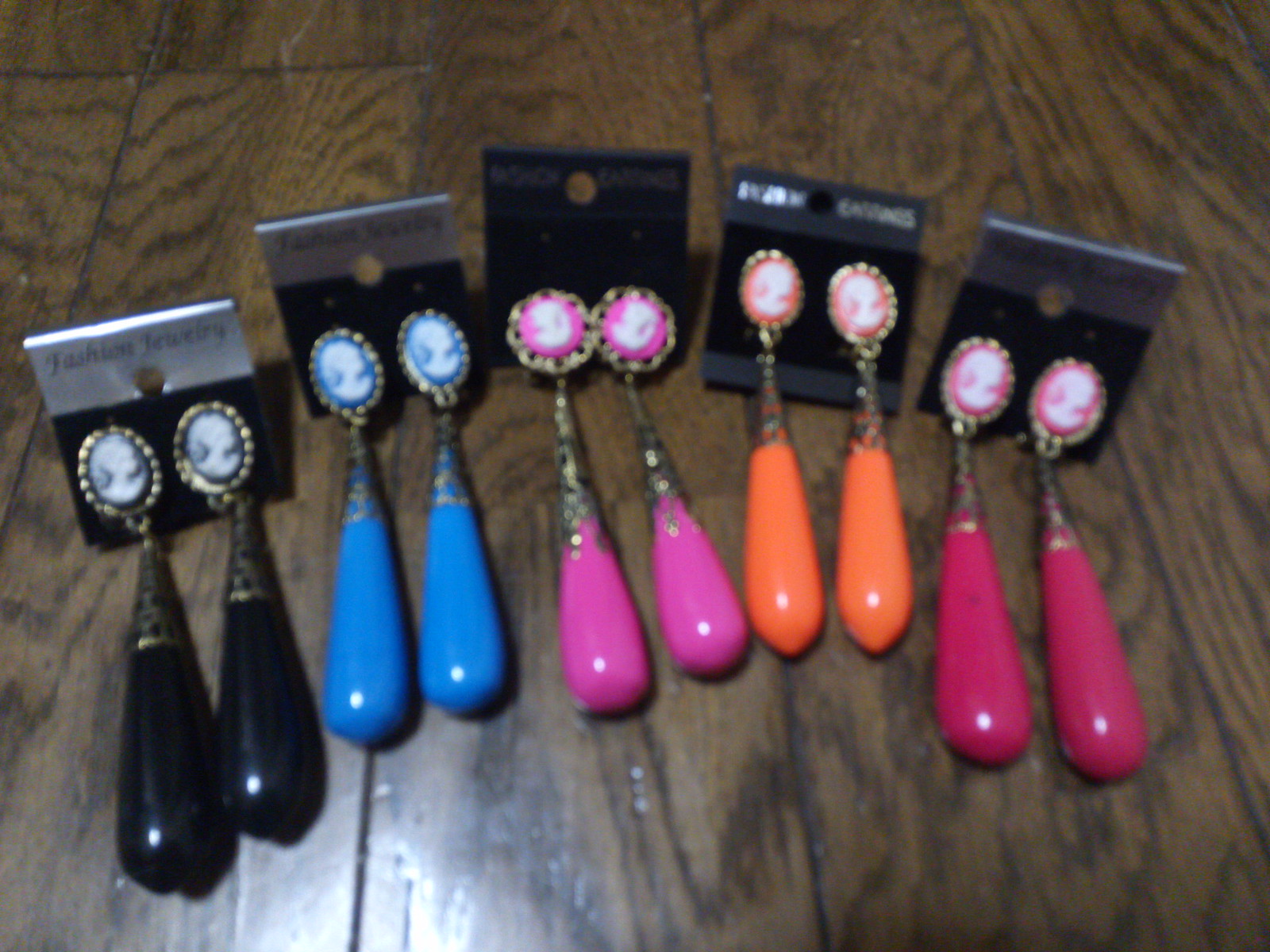The photograph features five pairs of similar earrings meticulously arranged on a table composed of dark wood planks. Each pair of earrings is attached to an identical packaging card made of cardboard or paper, punched with a hole at the top. The cards are distinguished by a silver upper half featuring the text "FASHION JEWELRY" in black, and a black lower half where the earrings are affixed. The earrings themselves all share the same elegant design: a round cameo portrait of a woman looking to the right, framed in gold, from which a large teardrop-shaped element hangs on a chain. The color of the cameo's background and matching teardrop differs for each pair, progressing from left to right in black, blue, pink, orange, and red. Despite some blurriness in the image, the overall layout and intricate detailing of the earrings' style are evident.